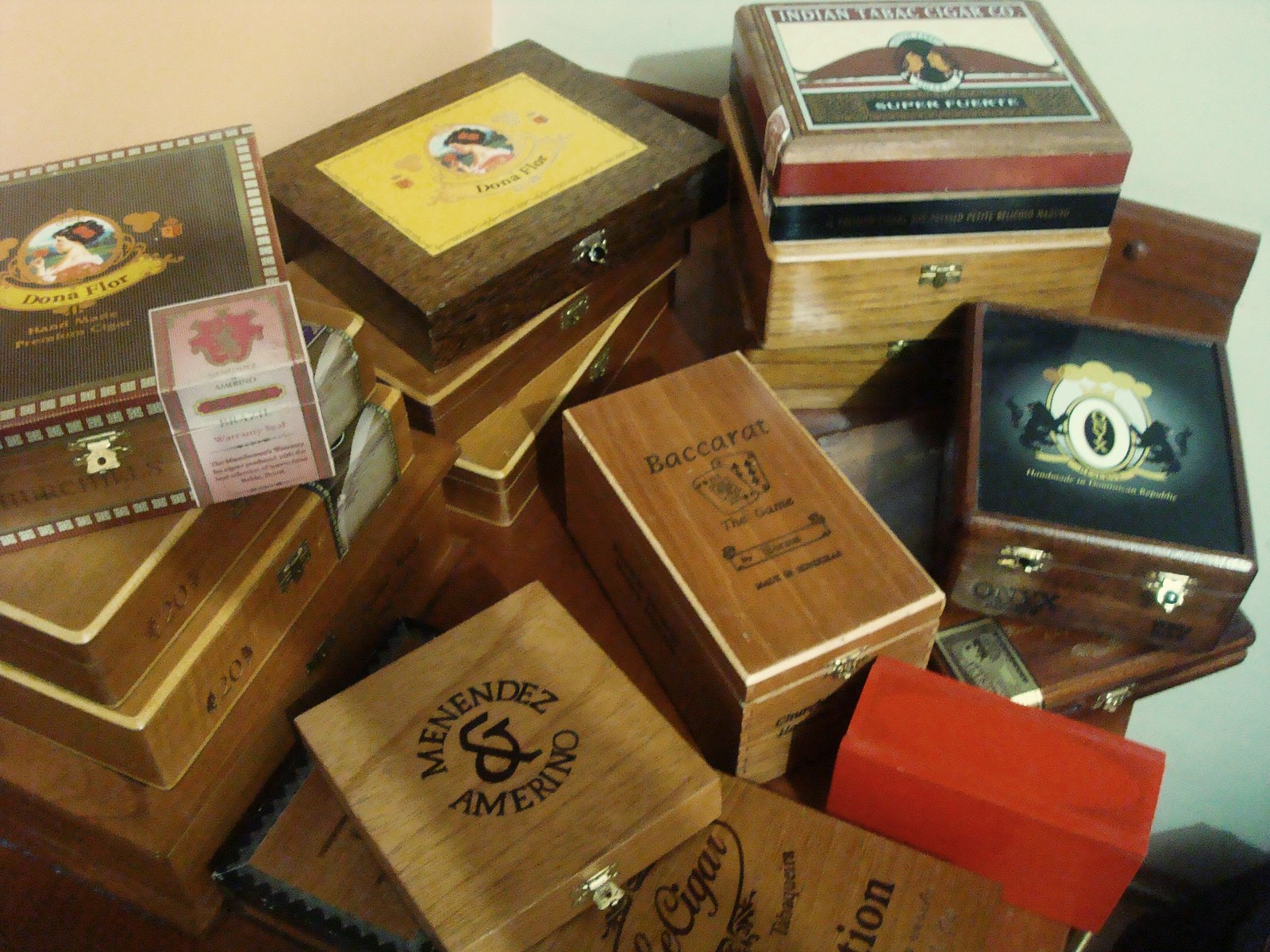The image captures a collection of 12 to 15 intricately decorated cigar boxes arranged on a table, with a detailed backdrop of a pale green wall on the right side and a tan wall on the left. Among the assortment, two prominent cigar boxes on the left side each feature a woman in a circle at the center, with an orange flower in her hair and a light brown dress draped over her shoulder, viewed from the left. The box on the left is primarily brown with a dashed white outline, while the one on the right has a yellow rectangular center framed by brown. Both of these boxes are stacked atop two additional brown boxes beneath them.

To the right, three more boxes are stacked vertically. At the top of this stack is a blue box adorned with silhouettes of lions reaching up to touch an oval. In the middle, there's a brown rectangular box branded with "Baccarat," and below it sits a red box with no visible writing. The entire collection includes various shapes and colors, with many boxes featuring chrome clasps, indicating they can be securely closed or locked. The front-most box visible in the lower right corner is marked "Menendez Amarino" in black lettering. The image is well-lit, highlighting the diverse designs and colorful details of the boxes while maintaining sharp focus throughout.